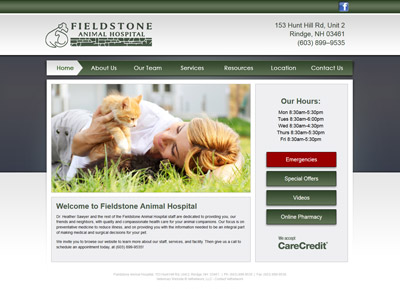The image showcases a vibrant and colorful website homepage for a veterinary clinic. At the top, there is a gray navigation bar with the Facebook logo, followed by the clinic's name, "Missionary Field Stone Animal Hospital." Below the header, a serene scene features a stone wall, a peaceful landscape, and a dog affectionately hugging a cat, embodying the caring and compassionate environment of the clinic.

The address of the clinic is prominently displayed as "153 Hunt Hill Road, Unit 2, Range, NH 03461," along with the contact number "603-899-9535." The navigation menu includes links to various sections such as "Home," "About Us," "Our Team," "Services," "Resources," "Kitchen," and "Contact Us."

Further down, the image depicts a woman lying on the grass next to a cat, and another person gently holding a kitten, reinforcing the clinic's commitment to animal care. A welcoming message highlights "Welcome to Missionary Field Stone Animal Hospital," and details the clinic's hours of operation: 
- Monday: 8:30 AM - 4:00 PM
- Wednesday: 8:30 AM - 4:00 PM 
- Thursday: 8:30 AM - 5:30 PM 
- Friday: 8:30 AM - 5:30 PM

A red bar features additional information about emergency services, special offers, videos, and the clinic's pharmacy. The image also indicates that the clinic accepts CareCredit, making pet healthcare accessible and affordable. Overall, the bright and cheerful design of the website evokes a sense of warmth and reliability for pet owners seeking veterinary services.